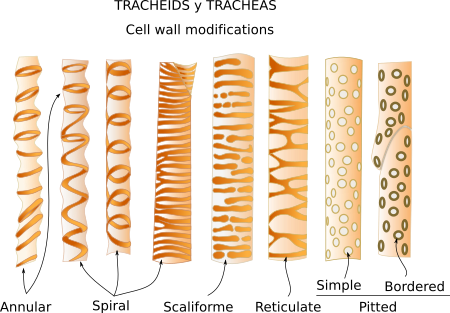The image is an informational diagram with a white background and black text titled "Tracheids etracheas Cell Wall Modifications." It features eight vertically aligned cylindrical depictions representing different types of cell wall modifications. The cylindrical figures are illustrated in light beige with darker beige patterns over them, accompanied by arrows highlighting specific structural details. Each modification is labeled at the bottom: 

1. **Annular**: Characterized by lines that go across, some angling up or down.
2. **Spiral**: Three columns, each with variations of spiral patterns; some curves make complete circles or loops.
3. **Scaliform (Scaliform)**: Displays horizontal lines with dashes.
4. **Reticulate**: Shows lines that create Y or H shapes across the surface.
5. **Simple**: Features small white dots scattered over the surface.
6. **Bordered**: Displays white dots with black outlines.

The detailed depiction and organized layout effectively differentiate each type of cell wall modification, providing clear visual references for their structural differences.